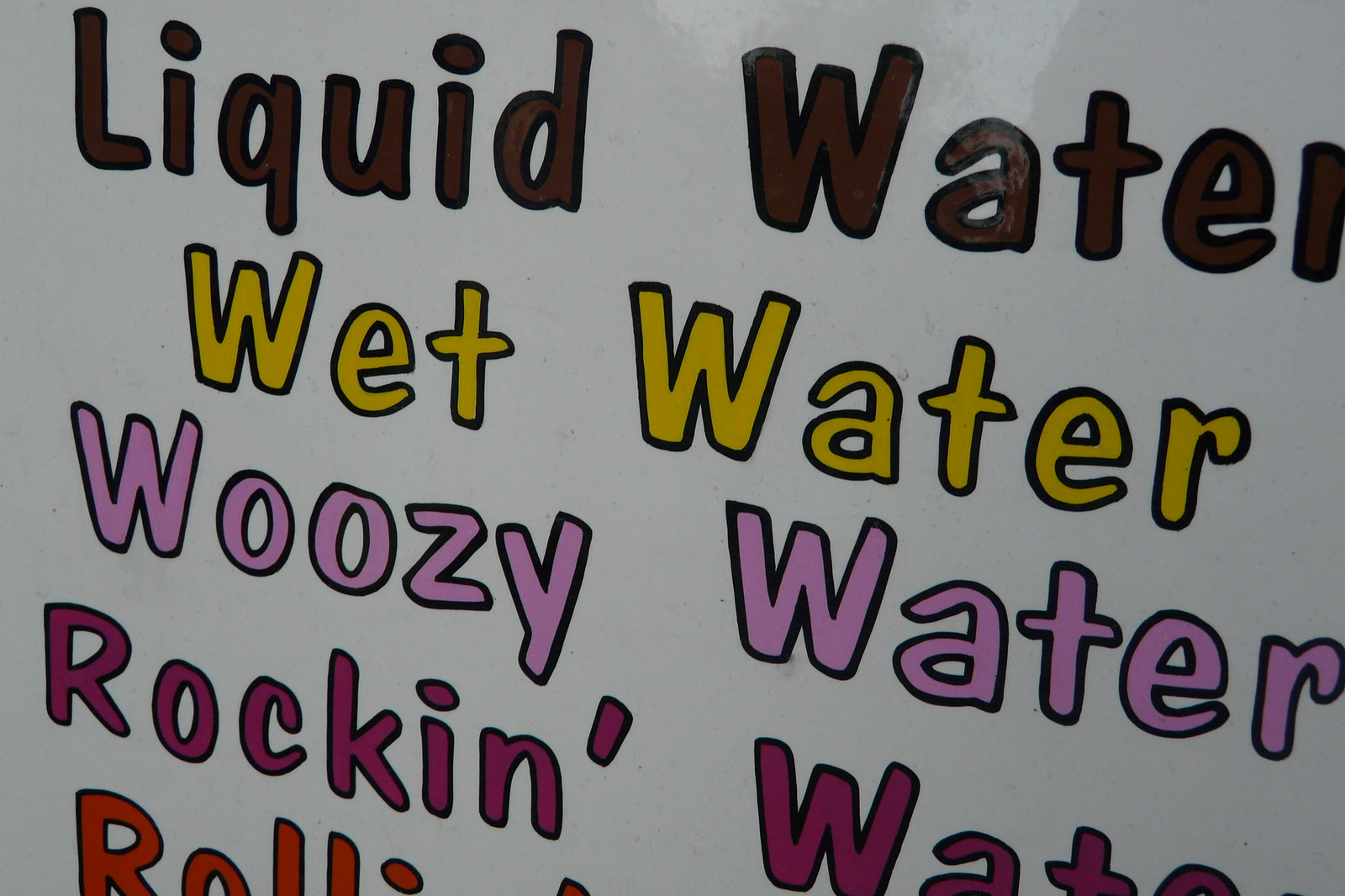This is a detailed close-up image of a potential car door or some sort of sign with a reflective metallic surface, indicated by a slight reflection in the top right corner typical of car paint. The image prominently displays multiple lines of text, each in different colored fonts with black borders. From the top, it reads "liquid water" in brown, "wet water" in dark yellow, "woozy water" in pink, and "rock and water" in red, though the letters "A," "T," and "E" are partially cut off. At the bottom left, only the word "rolls" in bright red is fully legible as the rest of this line is cropped from the image.